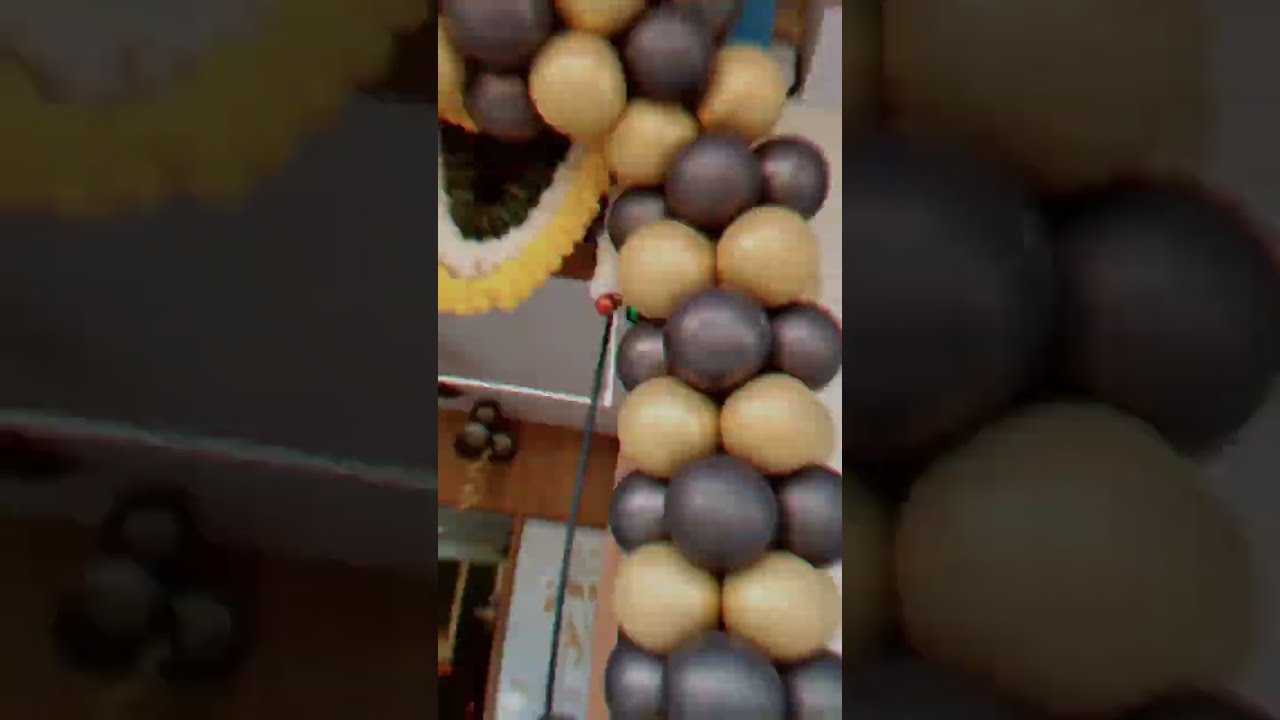The photograph depicts a tall, elaborate tower of balloons, resembling an arch, leaning against a wooden wall inside a building. The balloons come in various sizes and are arranged in alternating rows of grayish-black and brownish-gold hues, creating a striking visual pattern. Streamers in black, white, and goldish-yellow colors drape from the top of the arch, adding a festive touch. The floor beneath the balloons appears to be a smooth, hard surface, possibly hardwood, with some rugs nearby that feature brown with white stripes and white with peach accents. In the background, additional black balloons can be seen hanging from the ceiling. The central image is framed by zoomed-in, faded edges of the same scene, giving a sense of continuity and depth. The picture, with its rotated orientation and slightly fuzzy quality, captures the intricate details and muted lighting of the indoor setting.